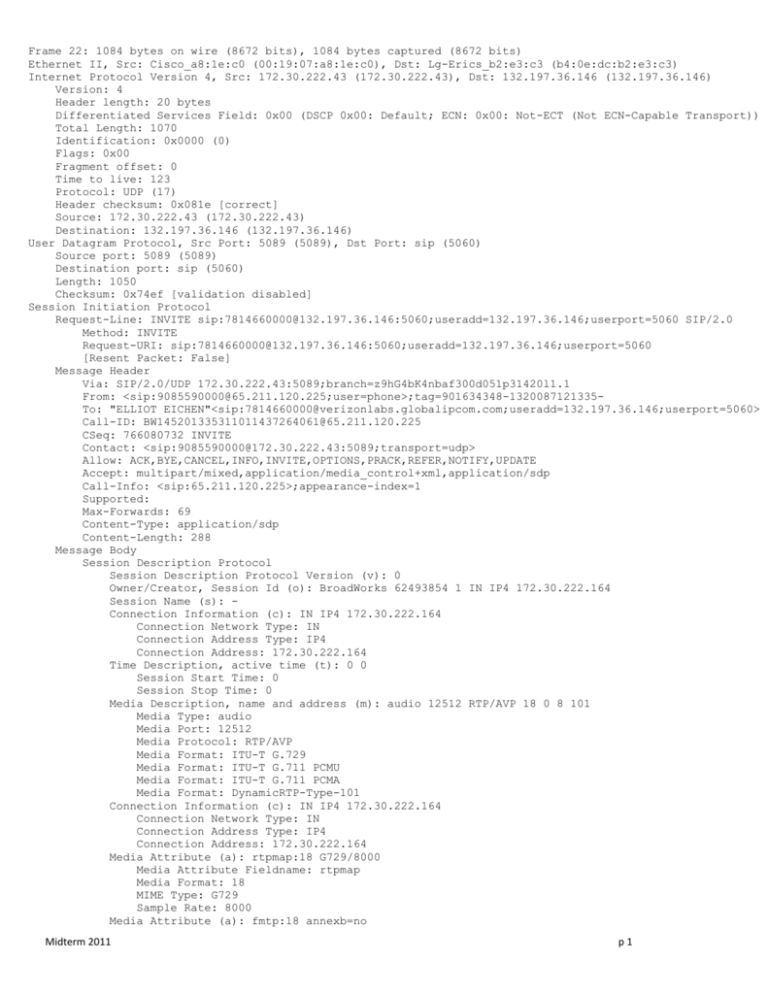This image features a white background with black text that resembles source code, potentially from a packet capture or protocol analysis output. The text begins with lines formatted as "Frame" followed by numerical identifiers, and it details various fields and parameters found in network communication protocols. Key elements include sections such as:

- **Ethernet II:** The data link layer protocol.
- **Internet Protocol Version 4 (IPv4):** Shows details like header length (20 bytes), total length (1070 bytes), identification code, flags, fragment offset, time to live, protocol, header checksum, source and destination addresses.
- **User Datagram Protocol (UDP):** Includes fields for source port, destination port, length, and checksum.
- **Session Initiation Protocol (SIP):** Provides details on request line, method, request URI, message header fields like via, from, to, call ID, contact, allow, accept, call info, supported, max forwards, content type (application), content length.

Additionally, there's information on the **Session Description Protocol (SDP):** Covering version, owner/creator, session ID, session name, connection information (network type and address), timing (active time, start time, stop time), and descriptions of media including media type, port, protocol, format, and attributes.

The content concludes at the bottom left corner of the page with a notation: "Midterm 2011," indicating that this might be related to an academic examination or a study material from that year.